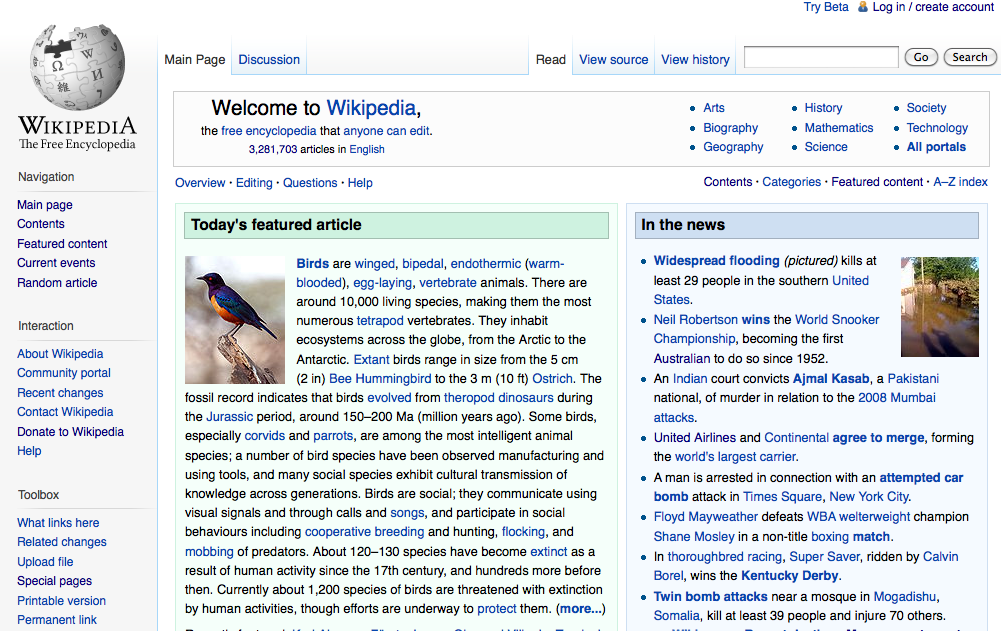Salam posted an image of the Wikipedia homepage. Wikipedia is an extensive online encyclopedia where users can contribute information on a vast array of topics. Despite being open to public contributions, edits are monitored and verified by dedicated contributors to maintain accuracy and credibility. Misleading or incorrect entries are corrected, and persistent offenders can be banned from editing.

The homepage, primarily designed with a white background and black text, features blue hyperlinks that direct users to additional pages on related topics. The current highlighted article focuses on birds. Additionally, the homepage includes a news section with updates on significant events, such as recent Westfield flooding and Robertson's World Snooker Championship. The layout is user-friendly, encouraging easy navigation through extensive information.